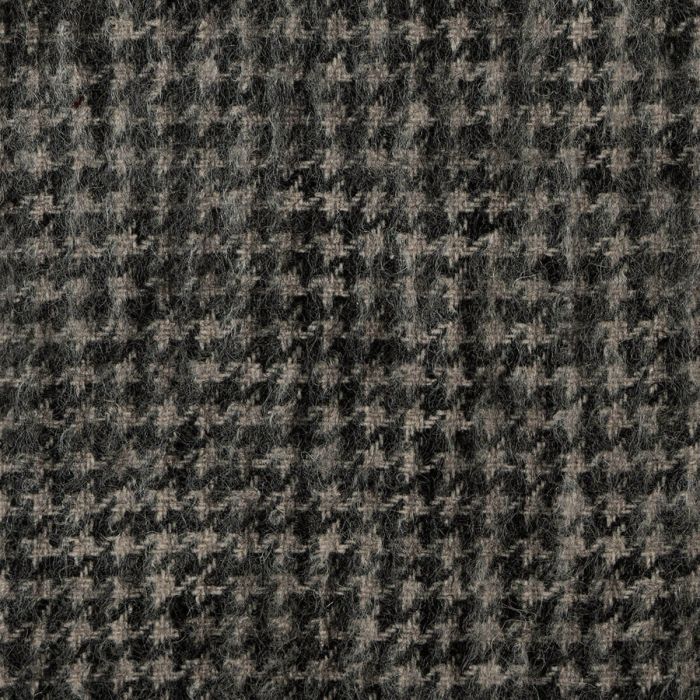This image depicts a highly zoomed-in view of a piece of fabric, revealing intricate and fibrous details. The fabric features a rigid texture and a pattern that may resemble houndstooth, consisting of small white elements set against a grayish-black background. However, due to the extreme close-up, the individual fibers and fine hairs within the fabric are prominent, making it challenging to discern the exact pattern or the scale of the object. The fabric could be part of a couch, a coat, a sweater, or possibly carpeting. The colors in the image appear to be in grayscale, with variations from black to different shades of gray, although some observers noted that there might be hues of dark green and khaki in the mix. There are no other objects visible in the image, keeping the focus solely on the texture and pattern of the fabric.